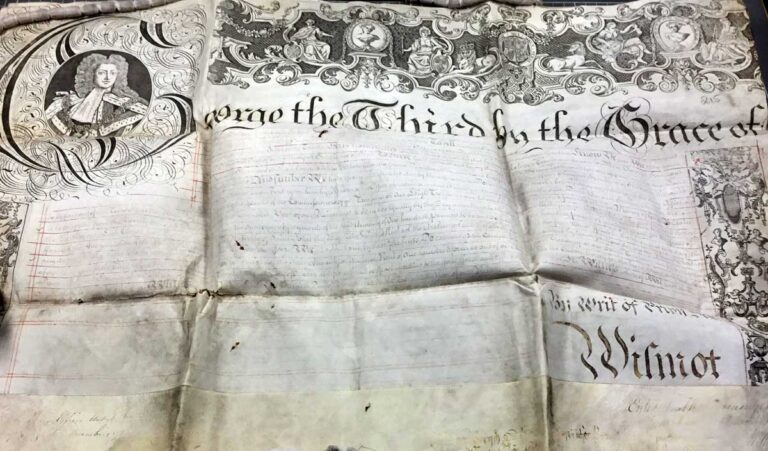The image showcases a very old, weather-worn document that has been unfolded and laid out. The document appears in black and white, with deep vertical and horizontal creases indicative of its age and wear. At the top, intricate designs depict scenes such as a carriage and people seated on thrones, reminiscent of Greek gods, as well as a unicorn. This area remains in fairly good shape compared to the rest of the document.

On the right side of the document is a portrait, likely of George III, characterized by long, frizzy hair and a dark jacket with a white scarf. The image is set within a circular frame and further encapsulated by a large letter "G." The document begins with the words "George III by the grace of" but the text following this is faded and partially illegible due to water damage and mildew. The overall degradation has caused much of the text to blur, making it difficult to discern the full contents of what appears to be some kind of decree. Additionally, the word "Wilmot" and phrases like "writ of" are somewhat legible towards the bottom right of the document. The background is mostly neutral with a small sliver of black at the upper right corner. The entire document conveys historical significance, suggesting its origin from the 1700s during the reign of George III, around the time of significant events such as the American Declaration of Independence.